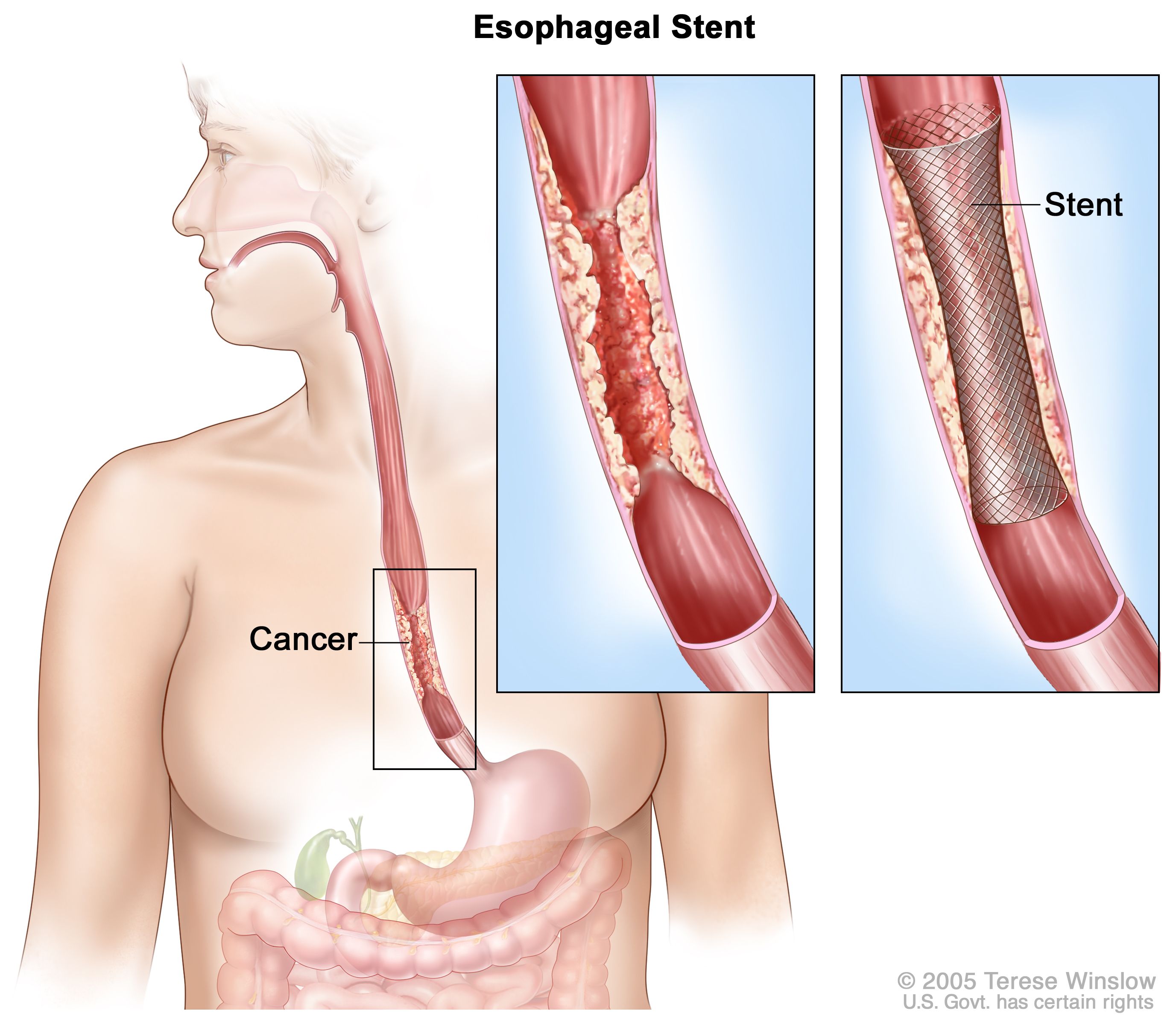This detailed medical diagram, sourced from a 2005 Teresa Winslow illustration with U.S. government rights, displays a step-by-step explanation of an esophageal stent procedure. The main illustration depicts a person facing forward with their head turned to the side, providing a transparent view of their internal anatomy. The esophagus, which extends down to the stomach, features a highlighted section near its base marked "cancer," showing a discolored, bumpy area indicative of the disease.

Adjacent to this primary depiction are two inset panels. The first panel offers a close-up view of the cancerous esophagus, demonstrating how the malignancy nearly blocks the passage, resulting in the damaged, strained tissue. The second panel illustrates the post-procedural state, where an esophageal stent has been employed to open up the narrowed space. This stent fortifies the weakened esophagus, ensuring the passage remains clear. 

Overall, the chart not only articulates the specifics of esophageal cancer and its impacts on the anatomy but also visually elaborates on how a stent can alleviate these blockages effectively.